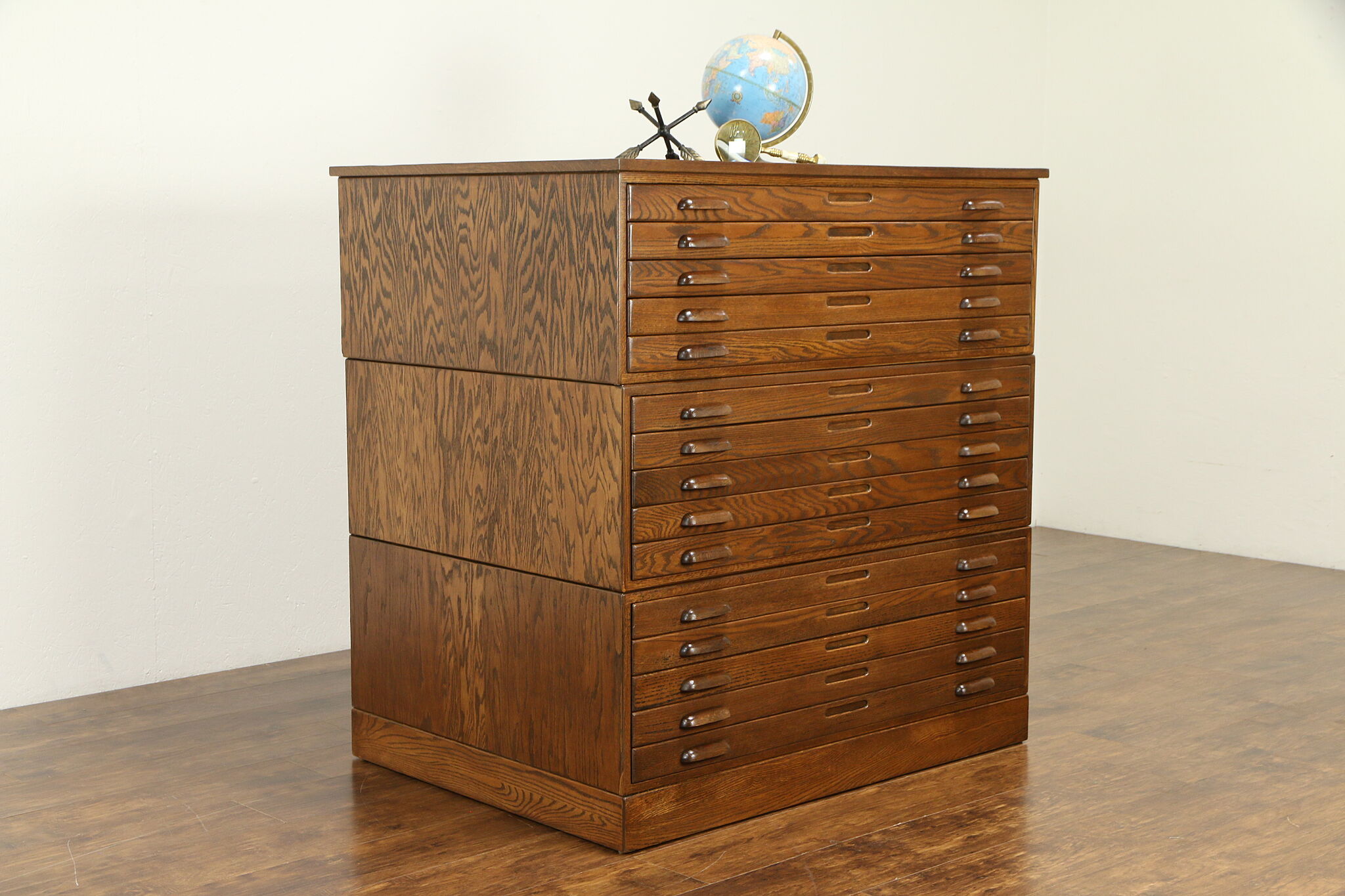In the image, an almost entirely empty room showcases a notable piece of furniture: a vintage wooden chest, characterized by its rich, dark brown color. This chest, likely an antique, stands against a white wall atop a shiny dark wood floor, adding to the room's simplicity and elegance. The chest is divided into three sections, each section containing five narrow drawers, making a total of 15 thin drawers, each equipped with handles on both ends. These drawers, possibly designed for storing small items or specimens, are neatly arranged in three rows of five. On top of the chest, a prominent globe with a gold axis, designed for easy rotation, shares space with a couple of intriguing metallic objects. To the right of the globe sits an upright metal object resembling a compass or an indicator, and beside it, a smaller, gold circular device with a rod extending from it, reminiscent of a weathervane. The minimalist setting highlights the detailed craftsmanship and curiosities resting on the chest.